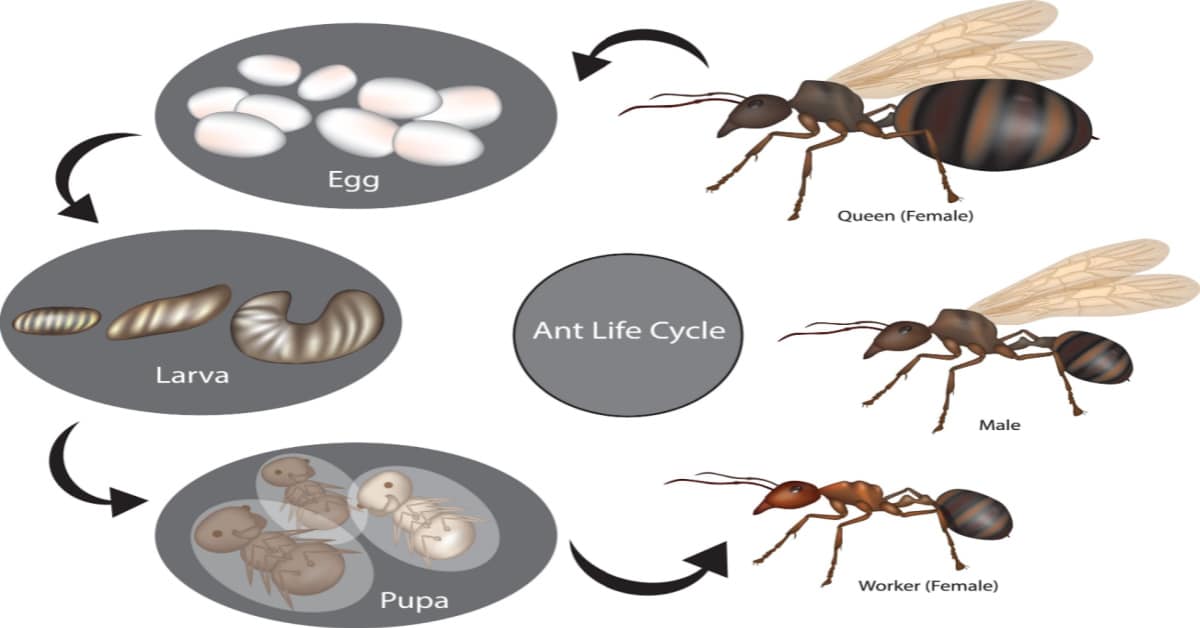This is a detailed poster depicting the life cycle of ants, presented with color illustrations against a black background. On the right-hand side, at the nine o'clock position, we see vertically aligned images starting with the queen ant at the top. The queen is illustrated in tans and browns with rings of black and is visibly larger with long wings. Below her is the male ant, also winged but smaller in size. Further down is the worker ant, identified as female, which lacks wings and is designed for ground work.

In the center of the poster is a large gray oval labeled "Ant Life Cycle" in white text. Arrows extend from the queen ant to various stages on the left-hand side, each stage enclosed within smaller gray ovals. The first oval, labeled "egg," depicts clusters of eggs. The arrow continues to the next oval showing these eggs developing into larva. Following this, another arrow points to the "pupa" stage, displaying the transitional phase where the larva transform into pupa. The final arrow leads back to the depiction of adult worker female ants, completing the cycle.

Overall, the poster intricately details the transformation from egg to adult ant, highlighting the significant roles and differences between the queen, male, and worker ants within the ant colony hierarchy.